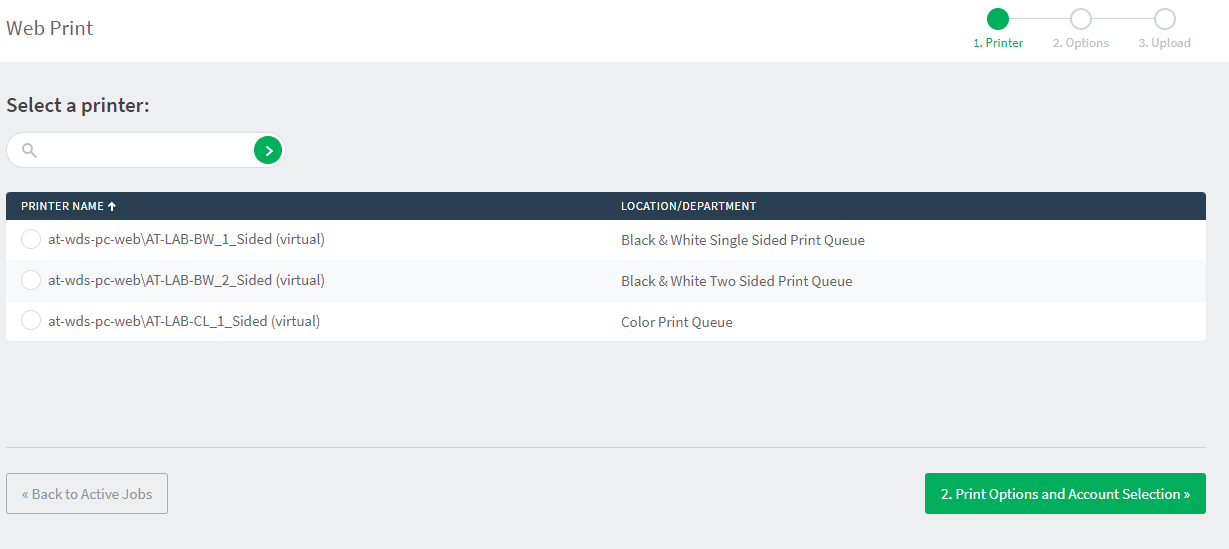This screenshot captures the web print interface. At the top left, the header "Web Print" is visible, flanked on the right by a three-step progress indicator comprising circles labeled "1. Printer," "2. Options," and "3. Upload." The "Printer" option is highlighted in green, indicating the current step.

Below the header, a gray box features the title "Select a Printer" on the far left. Adjacent to the title is a search field with a magnifying glass icon and a green arrow on the right side. 

In the section beneath this, a navy blue title bar labeled "Printer Name" and "Location/Department" appears. The list of available printers follows, alternating in white and gray backgrounds:

1. **First Option**: "AT-WDS-PC-Web/AT-LAB-BW_1_Sighted Virtual"
   - Description: Black and white, single-sided print queue.

2. **Second Option**: "AT-WDS-PC-Web/AT-LAB-BW_2_Sighted Virtual"
   - Description: Black and white, double-sided print queue.

3. **Third Option**: "AT-WDS-PC-Web/AT-LAB-CL_1_Sighted Virtual"
   - Description: Color print queue.

At the bottom of the screenshot, a grayed-out button labeled "Back to Active Jobs" is visible on the left, while on the right side, there is a button for "Print Options and Account Selection."